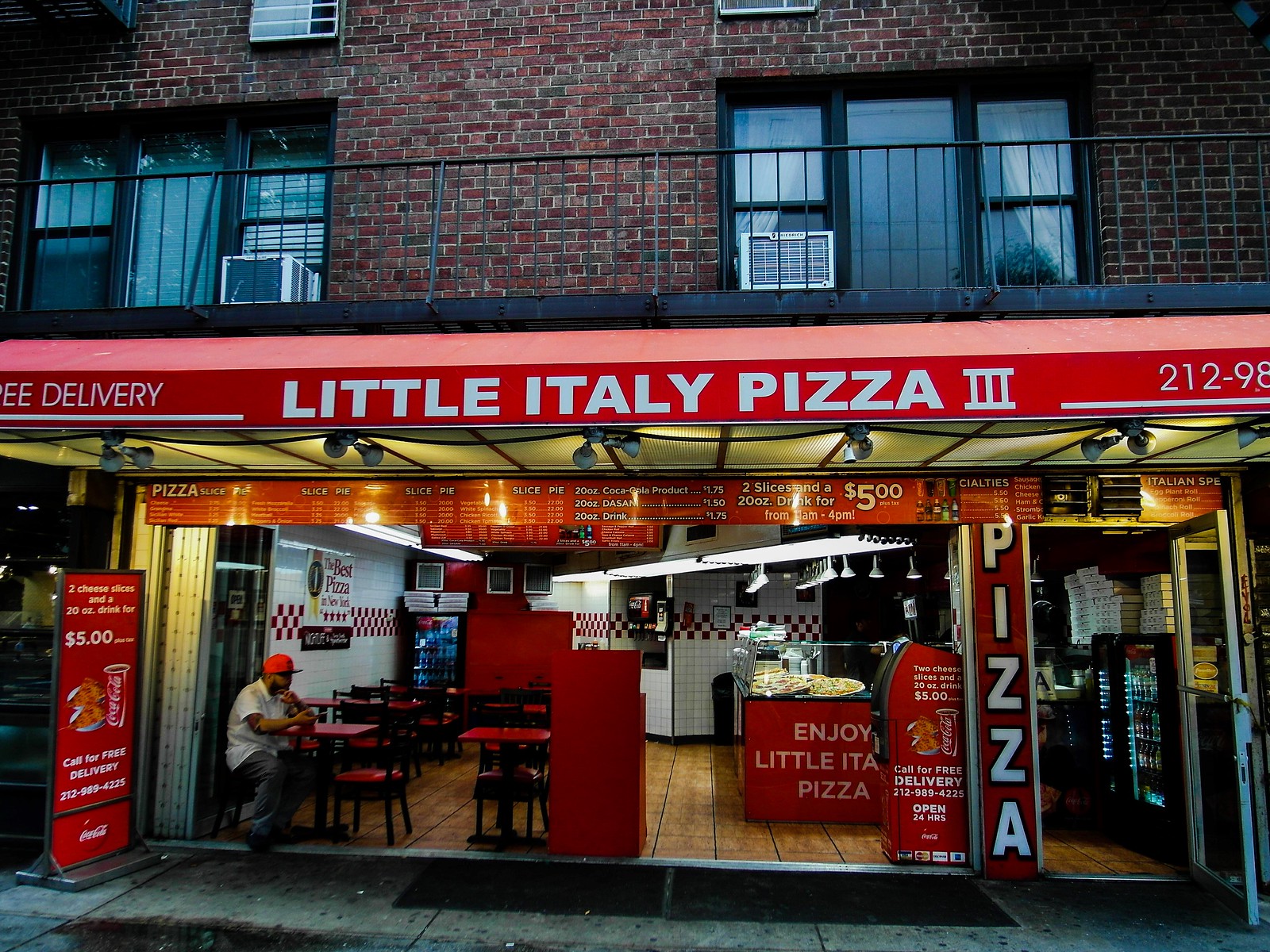The photograph captures the storefront of "Little Italy Pizza 3," located on the ground floor of a brick building with what appears to be residential apartments above, as evidenced by the window air conditioning units. The first floor features a red awning with white lettering that reads "Little Italy Pizza III" and includes a partial phone number beginning with "212-98." A sidewalk stand advertises a special promotion: two slices of pizza and a Coke for $5, along with free delivery.

Inside, the pizzeria is characterized by a combination of red and white decor, including red tables and chairs, and red and white tiles along the walls. A man in a red baseball cap sits alone at one of the tables, possibly indicating he works there. The interior also includes a glass counter showcasing stacked pizzas and a soda machine. Overall, the pizzeria exudes a welcoming, nostalgic charm that makes it a likely favorite in the neighborhood, despite the seemingly quiet moment captured in the photo.